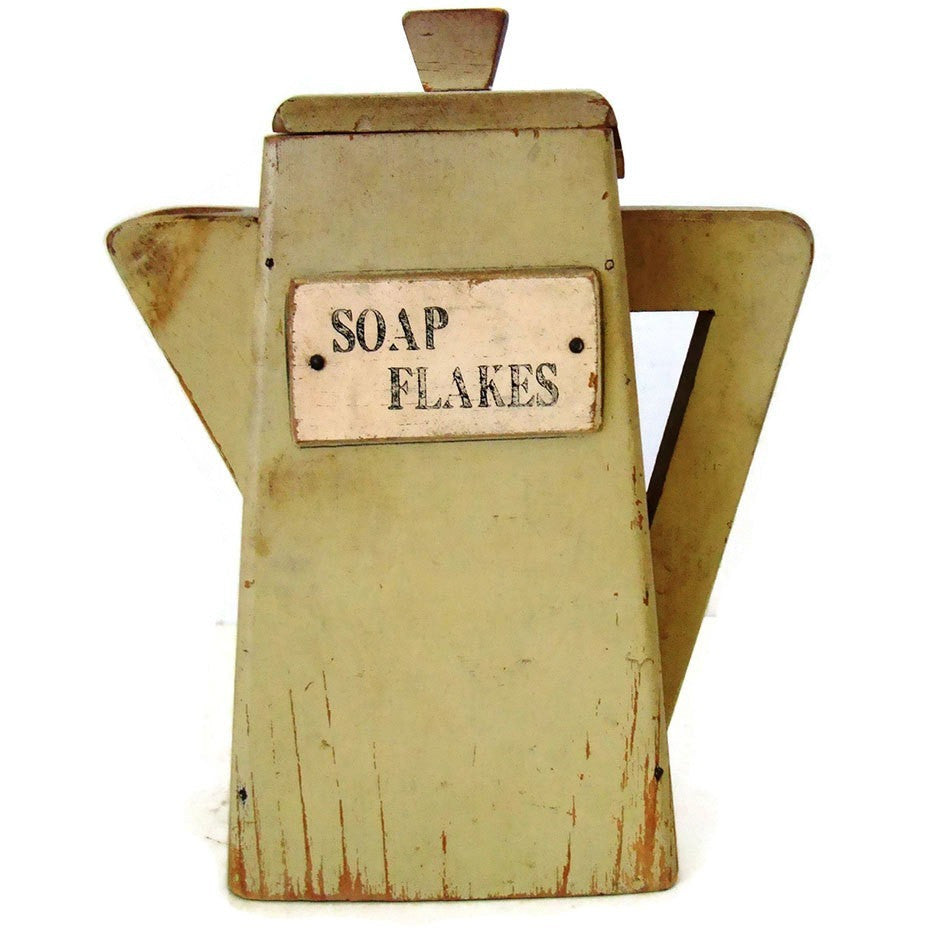This color photograph captures a vintage ceramic kettle-like container painted in a light brown or beige color, with darker brown streaks extending from the bottom towards the center, giving it an aged appearance. The container is cowbell-shaped, being wider at the bottom and narrower at the top. It features an angular design, with a triangular spout on the left and a right-side handle shaped like the number seven, straight along the length and curved at the top. The top of the container is fitted with a removable cap, which has a handle for easy lifting. Prominently displayed on the front is a pink rectangular label with black text that reads "Soap Flakes," the words "Soap" positioned at the top and "Flakes" at the bottom. The sign is affixed with two rivets and framed by a darker border, suggesting the container was intended to hold soap flakes. The entire setup rests against a plain white background, highlighting the intricate details of the container.